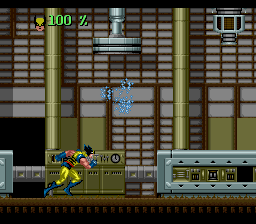This image is a screenshot from a pixel art, side-scrolling video game. The scene depicts the interior of a factory or industrial building, rendered in a compact frame. The character resembling Wolverine is visible at the bottom left, dressed in a yellow outfit with blue accents and sporting distinctive spiky black hair. The character is captured in mid-run, adding a sense of motion to the still image.

The background is composed of interconnected machinery, adorned with various buttons and symbols, intricately linked by an array of pipes. Two vertical pillars frame this mechanical backdrop, and a metallic wall with a grid-like pattern of small rectangles provides depth to the scene.

At the top-center of the image, a magnet-like apparatus is suspended from an arm affixed to the ceiling, emitting blue sparks that add a dynamic element to the environment. In the top left corner, the number "100%" is displayed alongside an icon of Wolverine's face, likely indicating the character's health or energy status in the game.